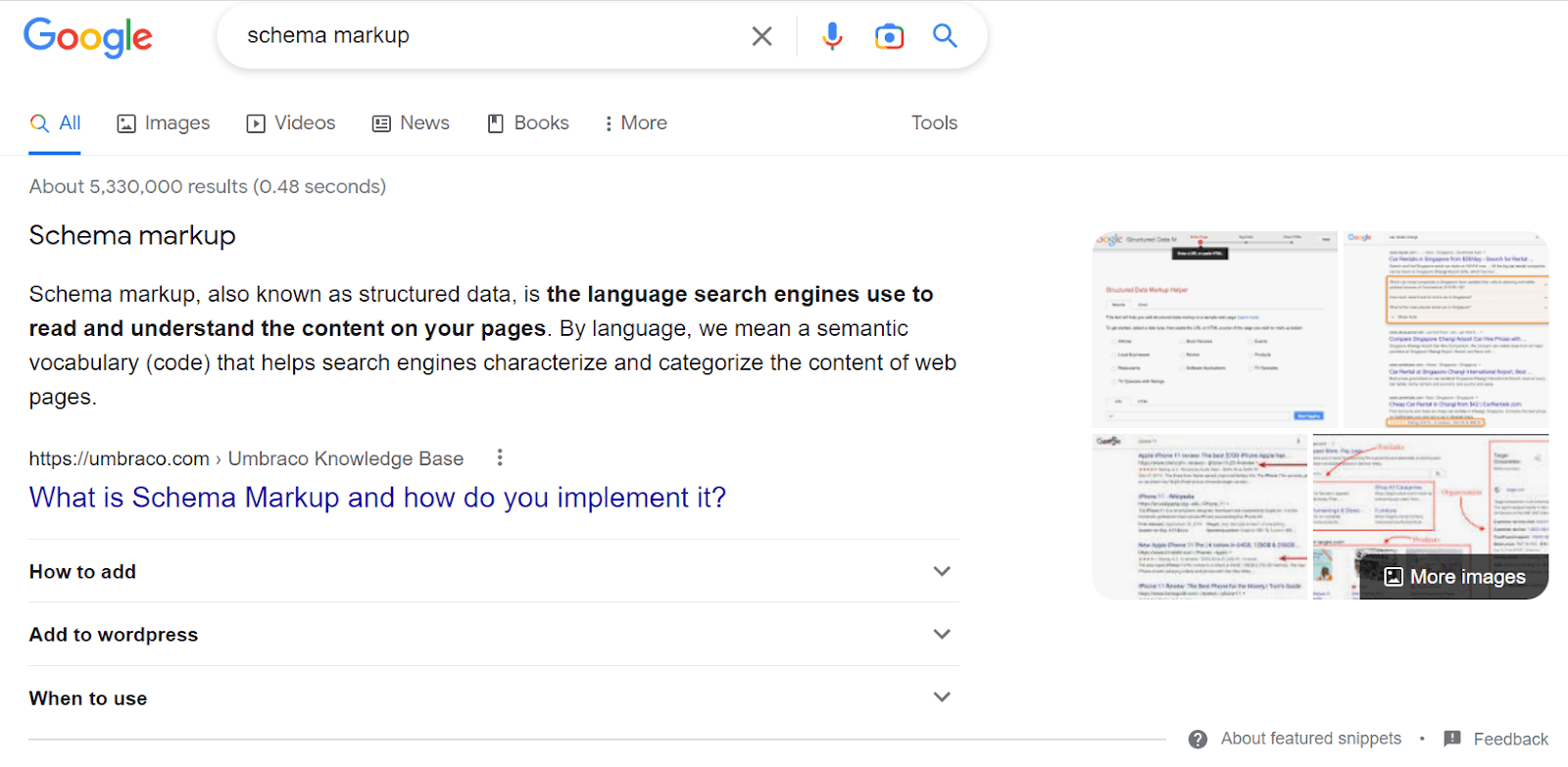The image depicts a detailed screenshot of a Google search results page. The top-left corner prominently features the Google logo, rendered in its distinctive blue, red, yellow, blue, green, and red colors. The search bar below the logo contains the query "schema markup," with an "X" icon to clear the search, followed by a microphone icon, a camera icon, and the search icon.

Directly beneath the search bar, a navigation menu offers various search categories, including "All," "Images," "Videos," "News," "Books," and a "More" option denoted by three dots, alongside the "Tools" button on the far right. This menu helps refine the search results.

Immediately under the menu, the page displays the total number of search results, "about 5,330,000," accomplished in "0.48 seconds". The primary search result is highlighted in bold text and reads "schema markup." The accompanying snippet explains, "Schema markup, also known as structured data, is the language search engines use to read and understand the content on your pages. By language, we mean a semantic vocabulary (code) that helps search engines characterize and categorize the contents of web pages."

Beneath this descriptive preview, the URL of the source website is listed, followed by a clickable blue hyperlink titled "What is schema markup, and how do you implement it?" This link takes users to the detailed article.

Further down, three additional dropdown results provide relevant subtopics: "How to add," "Add to WordPress," and "When to use." To the right of these dropdowns, there is an image thumbnail, presumably a screenshot, related to the first article result, enhancing the relevance and context of the search.

Overall, this screenshot offers a comprehensive view of the search results, showcasing Google's structured layout designed to provide users with easy navigation and quick access to pertinent information.